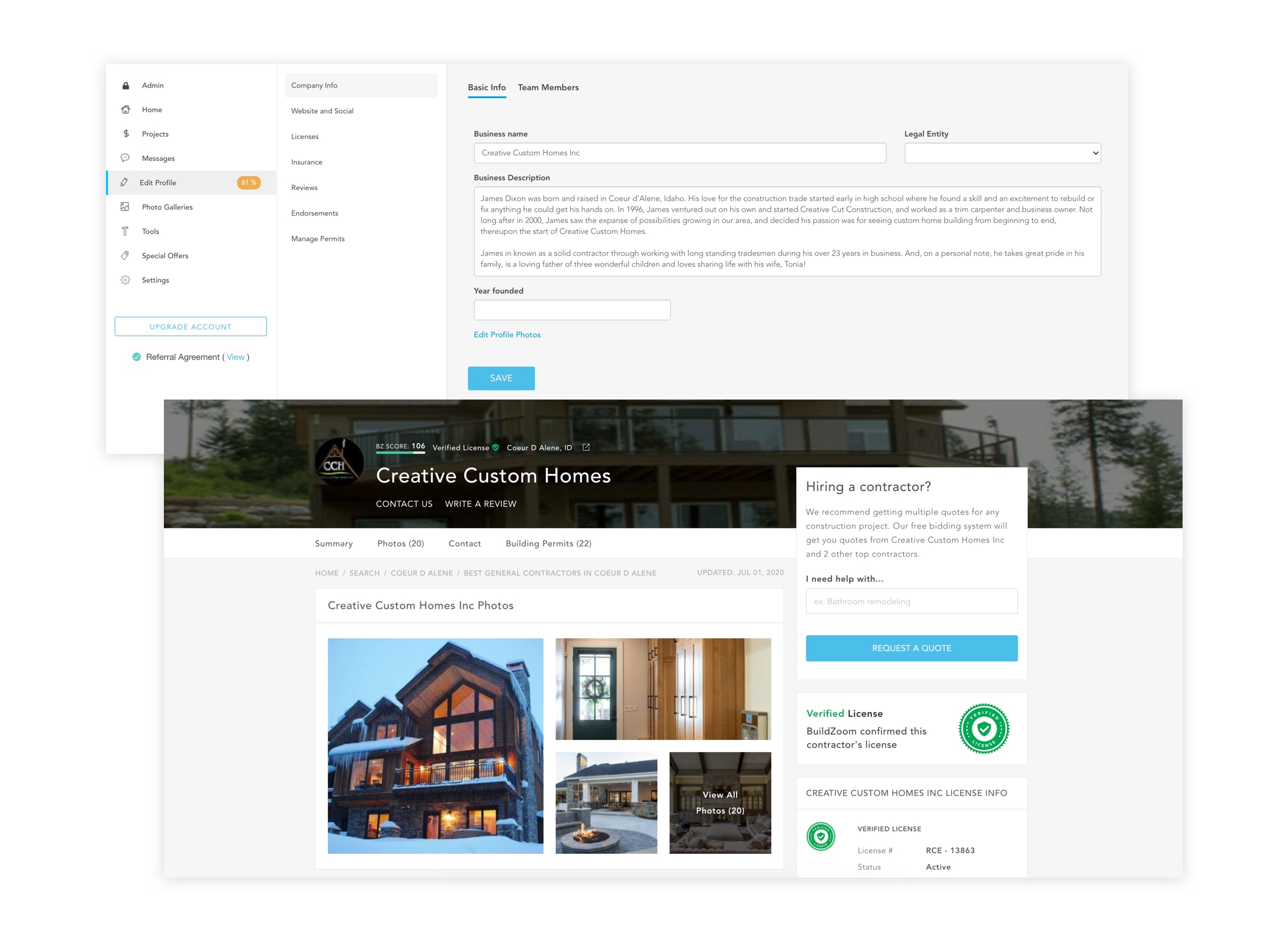This image comprises two overlapping horizontal screenshots, with the bottom one in the foreground.

### Top Screenshot (Background)
This background image primarily features a web page with a white and light gray theme. Two vertical toolbars with text run down the left-hand column. The main content area is divided into two sections: "Basic Info" and "Team Members." 

- **Basic Info Section:**
  - The "Basic Info" section is highlighted with a blue line.
  - Subsections include:
    - Business Name
    - Legal Entity
    - Business Description
    - Year Founded
  - A blue "Save" button is also visible.

- **Header:**
  - A translucent gray banner features a photograph of a house.
  - It says "Creative Custom Homes."

### Bottom Screenshot (Foreground)
This foreground image is a detailed webpage primarily about a specific construction project.

- **Header and Navigation:**
  - It includes four key headings: "Summary," "Photos," "Contact," and "Building Permits."
  - Below these headings, there is text that reads: "Home, Search, Koodaline, Best General Contractors in Koodaline, Updated July 1st, 2020."

- **Main Content:**
  - An editorial section about custom homes.
  - A large photograph of a snow-covered home on the left is accompanied by three additional detailed photos.
  - To the right is a vertical pop-up box with a white background that provides several options and pieces of information:
      - "Hiring a Contractor" heading.
      - A "I need help with" search term box.
      - A blue "Request a Quote" button.
      - A "Verified License" logo.
      - Subtitle: "Creative Custom Homes License Info."

This composite image provides a comprehensive overview of a web interface for managing business details and exploring contractor services, specifically tailored toward Creative Custom Homes, highlighting both navigation features and specific project details.